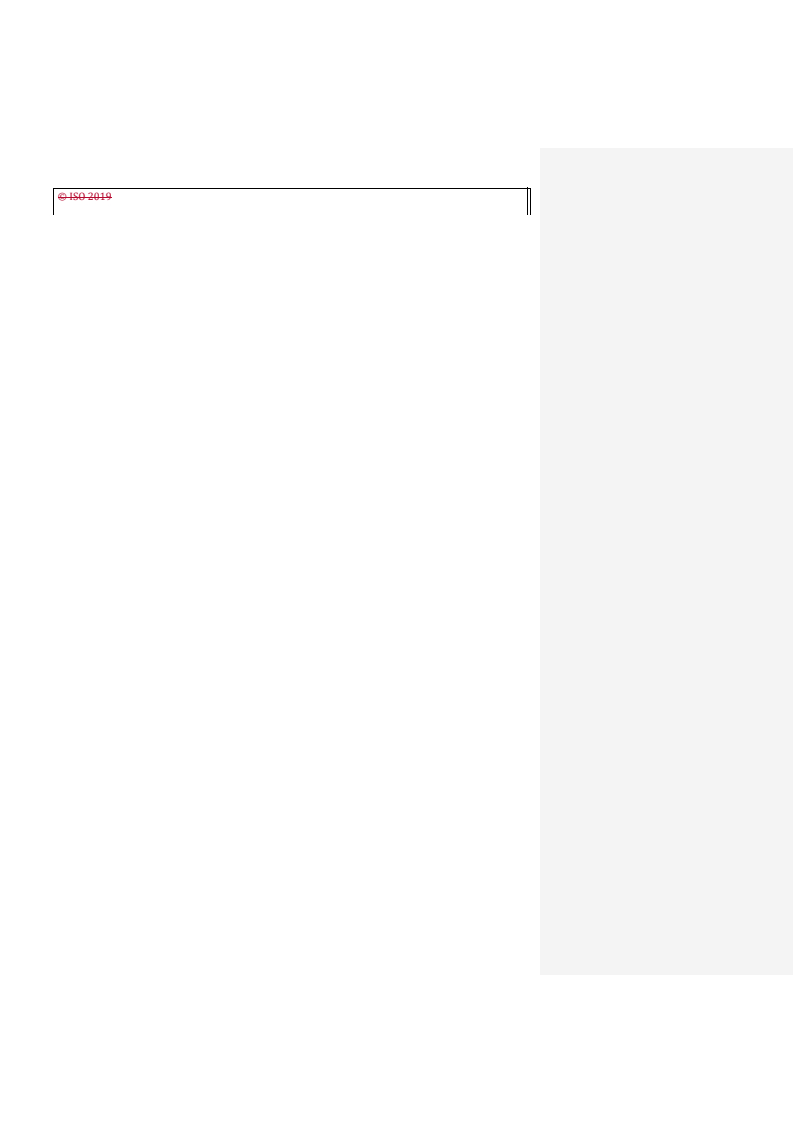The image depicts a horizontal black bar that spans from the left edge of the frame to approximately 75% of the image's width. The bar features slight downward extensions, or 'feet,' at both ends. Adjacent to the right end of this black bar is a slender, vertical gray box occupying around 25% of the image's width, extending from the top to the bottom of the frame. Inside the gray box, there is a red number with a line striking through it, accompanied by a small icon positioned nearby.